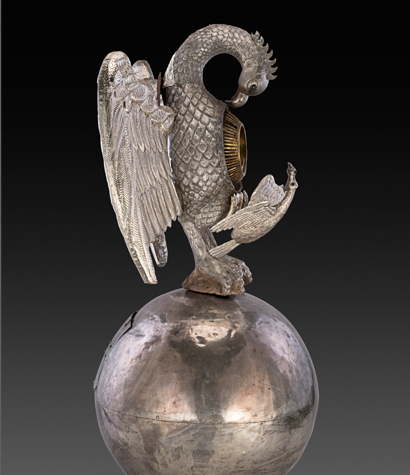The image captures a striking metallic statue set against a stark, dark gray background that transitions from black at the top to gray towards the bottom. The centerpiece of the statue is a majestic phoenix, distinguished by its mythical features. This mythical bird stands upright on a shiny silver sphere, displaying a body covered in intricate, scale-like feathers that gleam under the light. The phoenix's neck is gracefully craned downwards, resembling a hook, as it gazes at a smaller bird perched on its stomach. The smaller bird is secured by its tiny talons to a round, gold-colored indentation embedded in the phoenix's abdomen, adding a contrasting touch to the otherwise monochromatic statue. The larger bird's wings are elegantly spread out behind it, reminiscent of angelic wings, and faint spikes are visible along the back of its neck. Both birds, and the entire statue, exhibit a lustrous silver sheen that accentuates their detailed craftsmanship and reflects light beautifully. The dark gray background enhances the statue's metallic brilliance, creating a vivid and detailed visual spectacle.